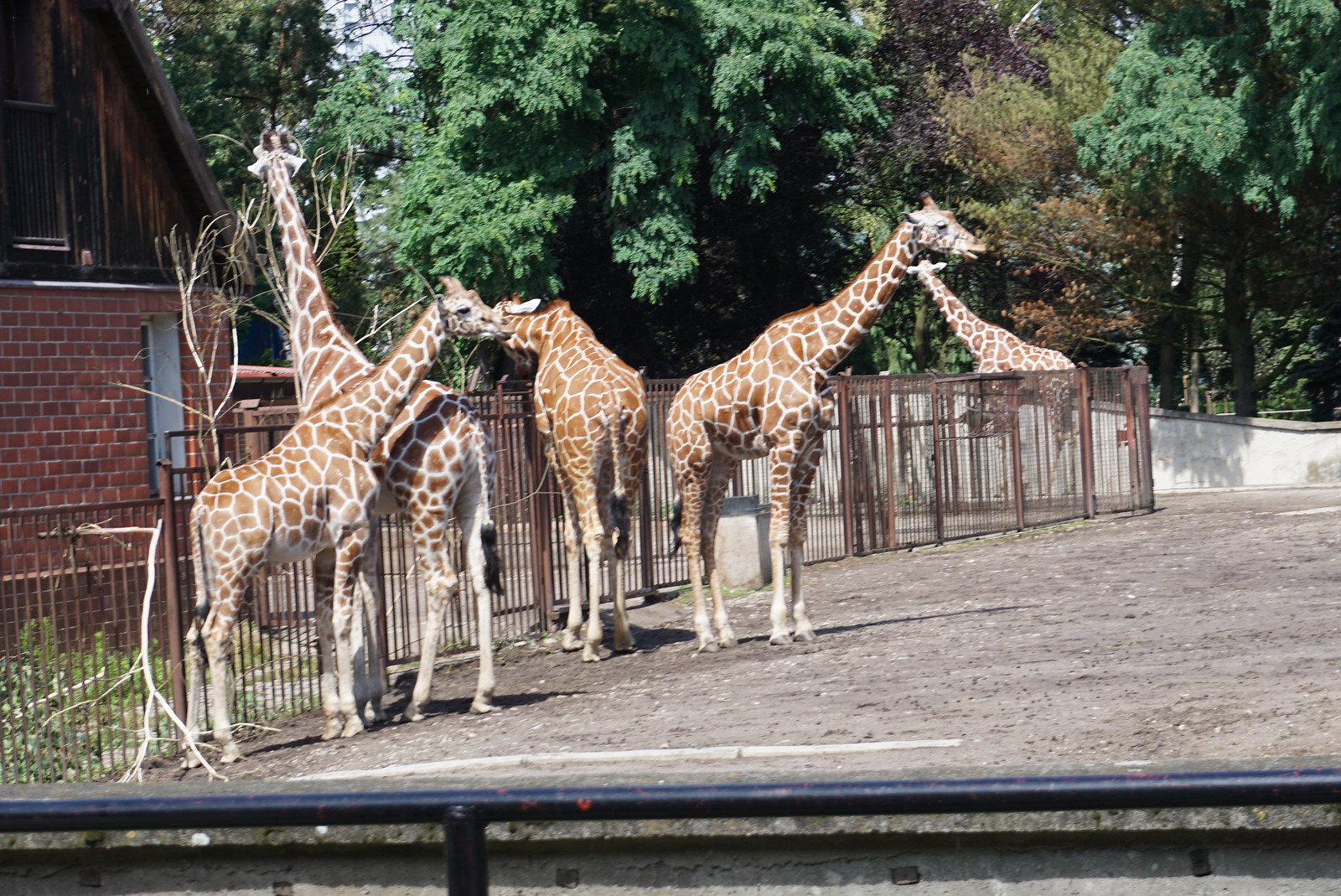A detailed photograph captures a tranquil zoo exhibit on what appears to be a sunny day. In the foreground, five giraffes, displaying their characteristic light brown circular spots with white lines, stand calmly on a mix of dirt and grey gravel ground. The giraffes are positioned in various orientations: two show their side profiles, another two display their backsides, and the fifth, farther in the background, looks off into the distance. Notably, one baby giraffe stands out, positioned in front of an adult and facing right, offering a clear profile view.

The habitat is enclosed by a fence transitioning from a rusted metal pole to black and then to a brown fence, which outlines the periphery of the exhibit. Beyond the fence, a picturesque backdrop of dark green trees occupies the upper third of the photo. On the left, partially overlapping the trees, stands a barn-like building with a red brick exterior base and a wooden roof. This building features a door and a window, adding architectural interest to the scene.

Adjacent to the fences are a series of iron cages containing branches, suggesting a form of feeding setup for the giraffes. This detailed and serene scene highlights the giraffes’ tranquil demeanor within a carefully constructed zoo habitat, complete with a mix of natural and man-made elements.